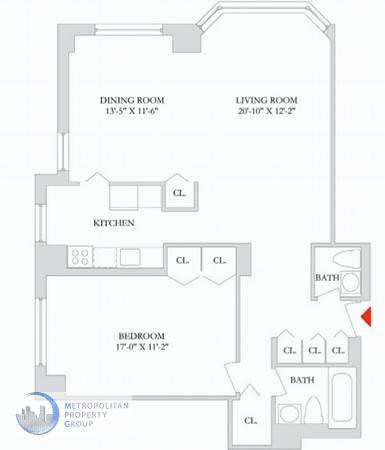This detailed floor plan represents a one-bedroom apartment managed by the Metropolitan Property Group, as indicated by the New York skyline silhouette at the bottom left of the document. The apartment—is compact yet well-designed, measuring a considerable 17 feet by 11.2 feet and is located on the bottom left corner of the layout. 

It features two spacious closets for ample storage and a private bathroom, accessible through a door at the bottom of the bedroom. Adjacent to this bathroom is a sizeable walk-in closet to the right, enhancing the storage space further. Additionally, three smaller closets are positioned straight through from this bathroom.

Adjacent to the bedroom is the kitchen, which seamlessly connects to a combined dining and living room area, forming an open and inviting space for relaxation and entertainment. Continuing straight from the living room towards the kitchen, one encounters an additional bathroom situated on the left-hand side, conveniently located near the apartment’s main entrance. This thorough description captures the thoughtful layout and space utilization of this one-bedroom unit, ideal for urban living.